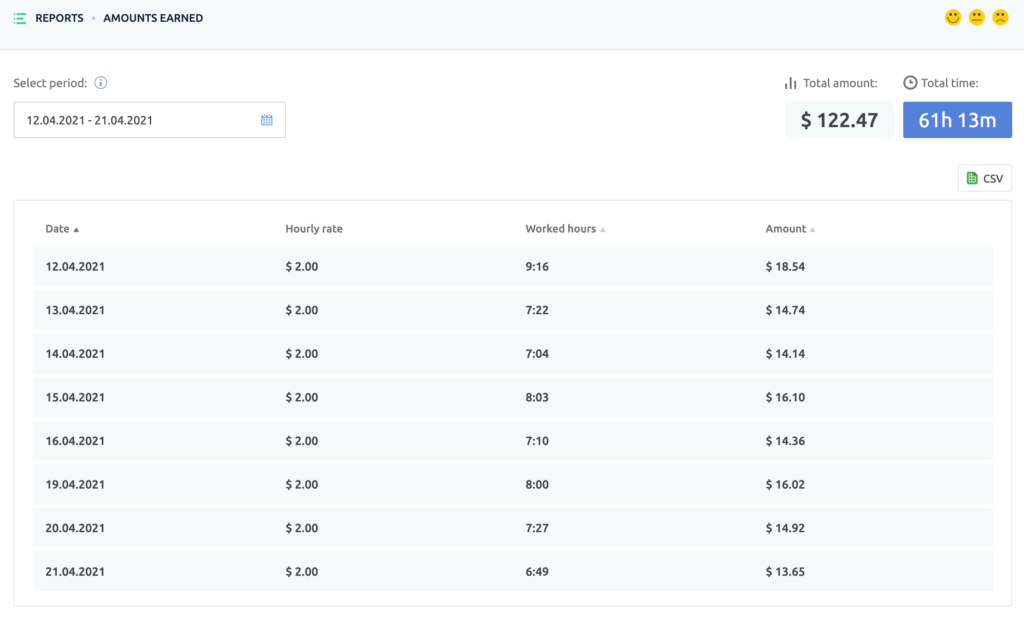The image features a detailed report on a white background. At the top, there is a light blue box with three small blue lines labeled "Reports and Amounts Earned," which includes three smiley faces representing different satisfaction levels: a happy face, a neutral face, and a frowning face.

Below this, there is a selectable date range box displaying "12/04/2021 to 21/04/2021" with a small calendar icon. This section is outlined in a slightly darker blue box.

Further down, there are statistics in a blue box showing the total amount earned as $122.47, displayed in a light blue subsection, and the total time worked as 6 hours and 13 minutes.

The main content consists of a table with headers in white: "Date," "Hourly Rate," "Worked Hours," and "Amount." The detailed breakdown is as follows:

- 12/04/2021: $2.00/hr, 9.16 hours, $18.54
- 13/04/2021: $2.00/hr, 7.22 hours, $14.74
- 14/04/2021: $2.00/hr, 7.04 hours, $14.14
- 15/04/2021: $2.00/hr, 8.03 hours, $16.10
- 16/04/2021: $2.00/hr, 7.10 hours, $14.36
- 19/04/2021: $2.00/hr, 8.00 hours, $16.02
- 20/04/2021: $2.00/hr, 7.27 hours, $14.92
- 21/04/2021: $2.00/hr, 6.49 hours, $13.65